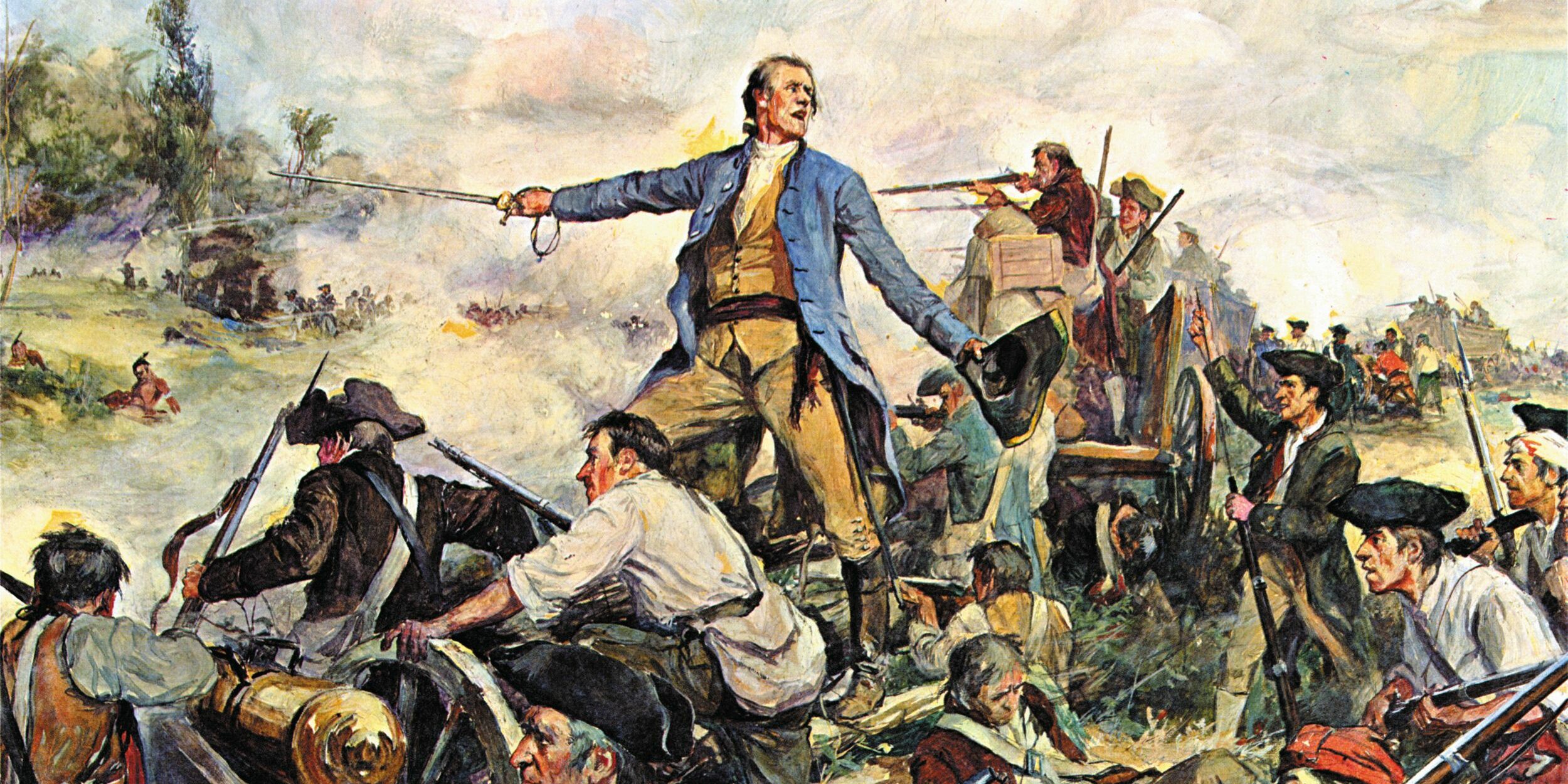The painting depicts a wartime scene, likely from the 17th or 18th century, featuring a group of European soldiers dressed in period attire, including long coats, tri-corner hats, pants, and suits. The central figure, an older man with grayish-brown hair, distinguished by his blue jacket, yellow vest, and yellow pants, stands prominently in the middle holding a black tri-corner hat in his left hand and a sword in his right. He appears to be a commander, directing his troops who are primarily situated on the right side of the image. The soldiers are engaged in battle, aiming and firing muskets and shotguns, while others wield swords. The background reveals ships and additional men, depicted in smaller sizes to convey distance. To the left of the image, trees and vegetation are visible, with some elements suggesting the presence of hidden enemies or Native Americans. The leader's dynamic pose, pointing and shouting commands, captures the intensity of the daytime confrontation, underscoring the chaos of the scene.